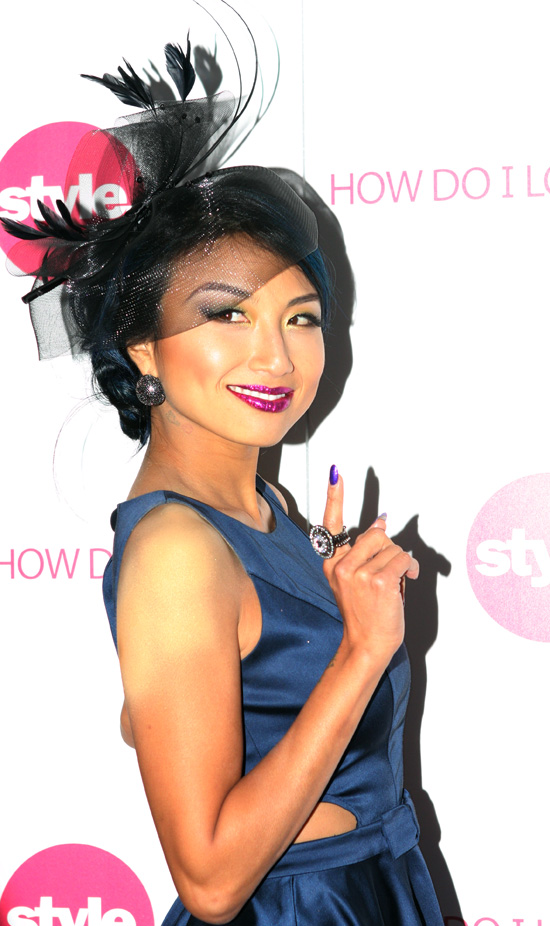In this striking image, a stylish woman is captured posing elegantly, dressed in a sleeveless dark blue dress with a revealing cutout just above her hip. The dress, shimmering under the lights, complements her dark blue nail polish. She holds her right hand up, with her index finger pointed straight up, showcasing a large, sparkly black ring. Her dark, short, and poofy hair is adorned with a chic black headpiece featuring feathers and black tulle, adding to her sophisticated look. Her makeup is bold, with dark, thick eye makeup and a striking dark red lipstick. The woman’s head is turned slightly to the side as she smiles, not directly at the camera, hinting at multiple cameras capturing her. Behind her, a white backdrop is decorated with alternating red circles and text reading "style" and "how do I look," emphasizing the fashionable theme of the scene. Black earrings, matching her ring, further enhance her ensemble.